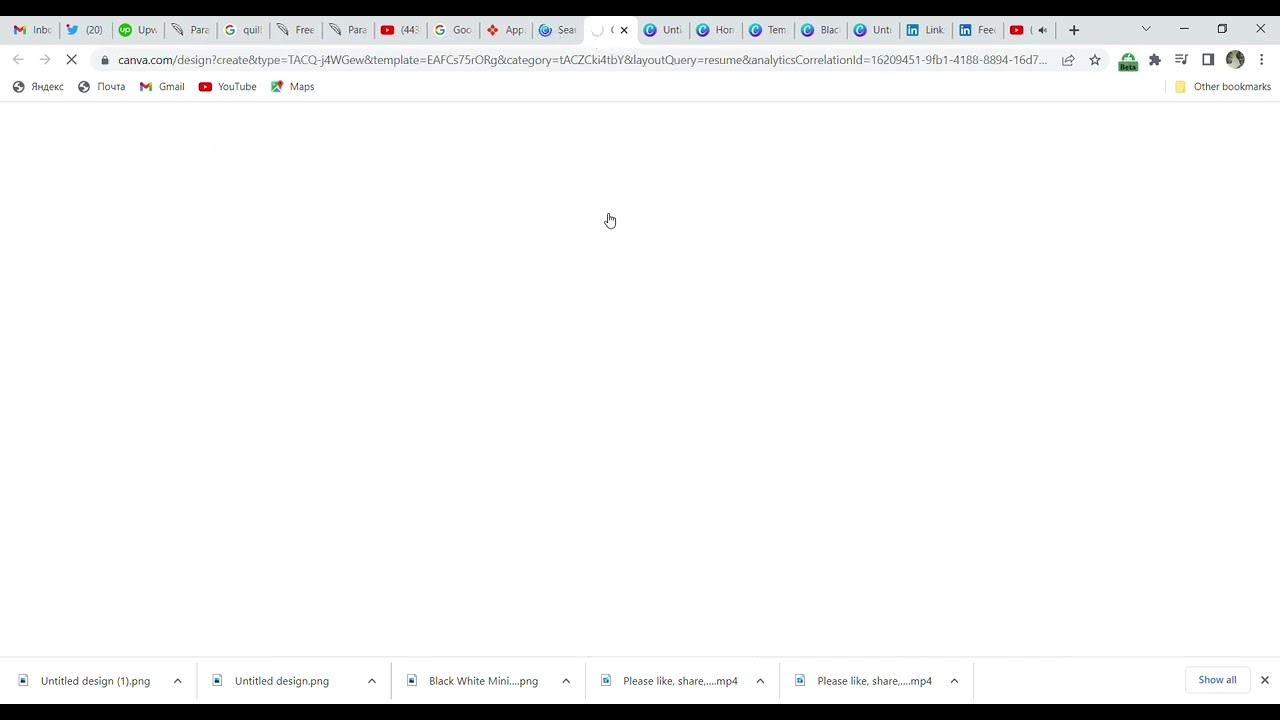This image is a detailed screenshot of a high-definition Chrome browser window. At the very top, the browser's tab bar is densely populated with approximately 20 to 25 open tabs, including Gmail, YouTube, Maps, Twitter, Upwork, Google, LinkedIn, and multiple instances of YouTube and Google. The currently active tab is trying to load a page on Canva.com, which involves creating a design. Directly below the tab bar is a prominent address bar showing the Canva URL, although the page itself remains blank and white as it is still loading. Below the address bar is the bookmarks bar, featuring shortcuts to various frequently used sites such as Gmail, YouTube, and Maps. At the bottom, there's a horizontal bar indicating several downloaded files, specifically untitled designs. The image is framed by two thin black horizontal strips at the top and bottom, which are part of the computer screen's border. A small hand cursor is visible, indicating the mouse’s position.